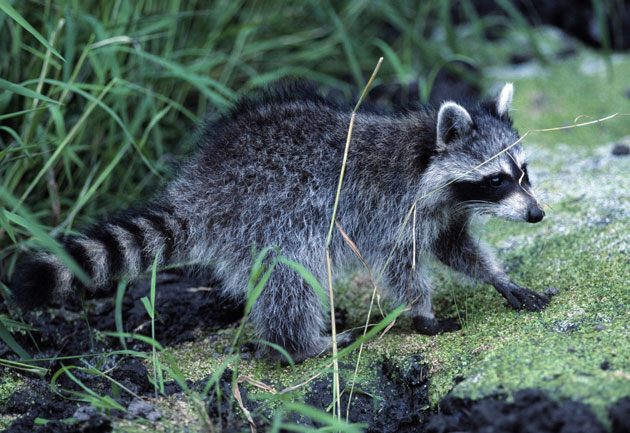The image captures a close-up side view of a young raccoon walking outdoors, likely in a forest or zoo setting. The raccoon, characterized by its distinctive black-and-white fur, is seen in full stride on what appears to be a moss-covered rock. Its fur exhibits a mixture of gray, black, and white tones, with a particularly striking black mask around its eyes and white fur above its eyes and nose, giving it the appearance of wearing a mask. The ears are also a mix of black and white, and its black paws stand out against the greenery. The tail has clearly defined black and grayish-white stripes. In the background, there is an abundance of greenery, including tall, thin grass, adding a natural and serene feel to the setting.